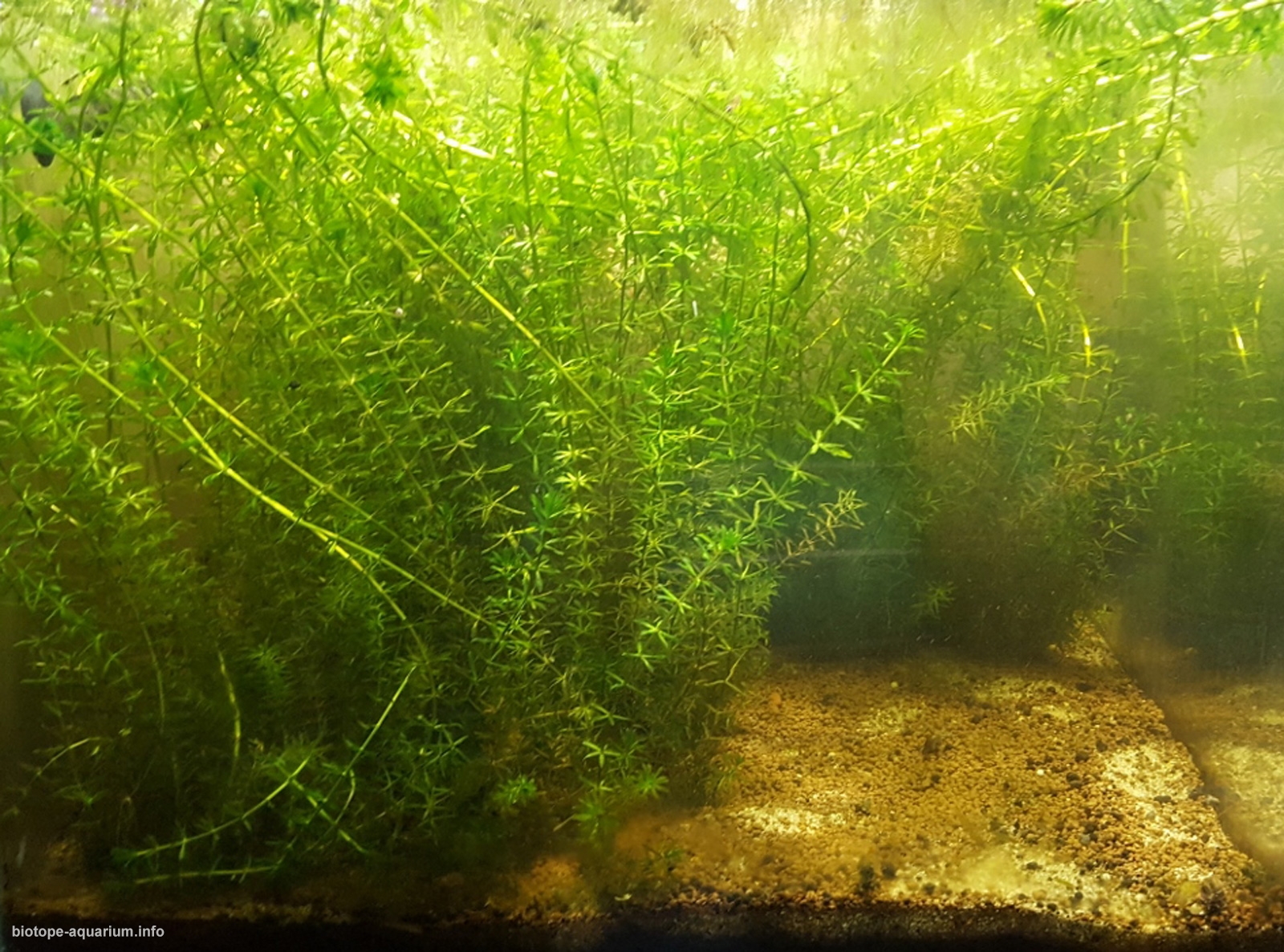This image shows the inside of an aquarium illuminated by an overhead light source, the nature of which is indeterminable. Predominantly occupying the left side and most of the image is a lush, dense arrangement of green aquatic ferns with slender leaves. These ferns, common in aquariums, create a vibrant yet somewhat muddled scene, indicative of either clouded water or potential organisms within it. The sandy bottom of the tank is visible on the right, making a sharp contrast with the greenery. Notably, the bottom left corner of the image features a piece of white tape inscribed with "biotope-aquarium.info," suggesting the origin of the photograph. Scattered throughout the scene are black seed pods, adding further detail to the diverse aquatic plant life.